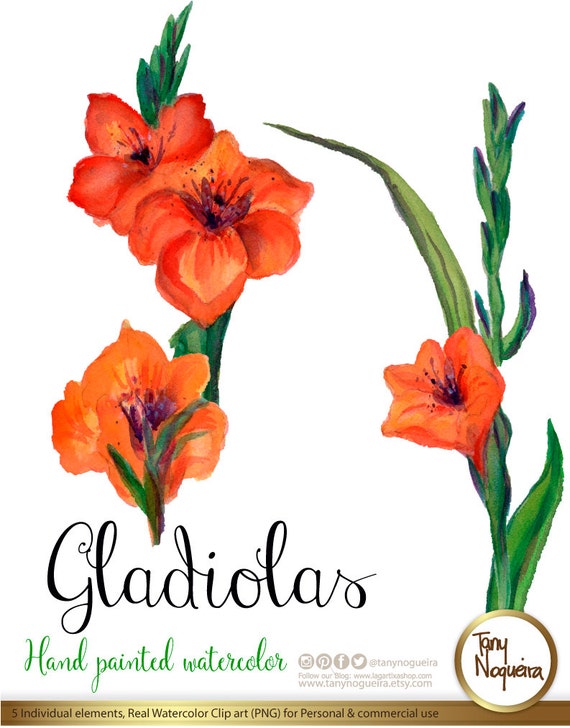The image is a clipart illustration of four orange gladiolus flowers attached to green stems, rendered in a hand-painted watercolor style. The composition features three sets of flowers: one plant with three orange gladiolus flowers, another with two, and a tall green stalk on the right with a single orange gladiolus. The text embedded in the image reads, "Gladiolus, hand painted watercolor," followed by the artist's name, "Tanynoguera," and a call to follow their blog at www.tanynoguerashop.com and www.tanynoguera.etsy.com. In the bottom right corner, there is a gold circle containing the artist's name "Tanynoguera" in cursive. Below this, a gold band stretches across the bottom with the text "Five individual elements, real watercolor clipart, PNG for personal and commercial use" written in black. Icons for social media platforms such as Facebook and Instagram are also present.